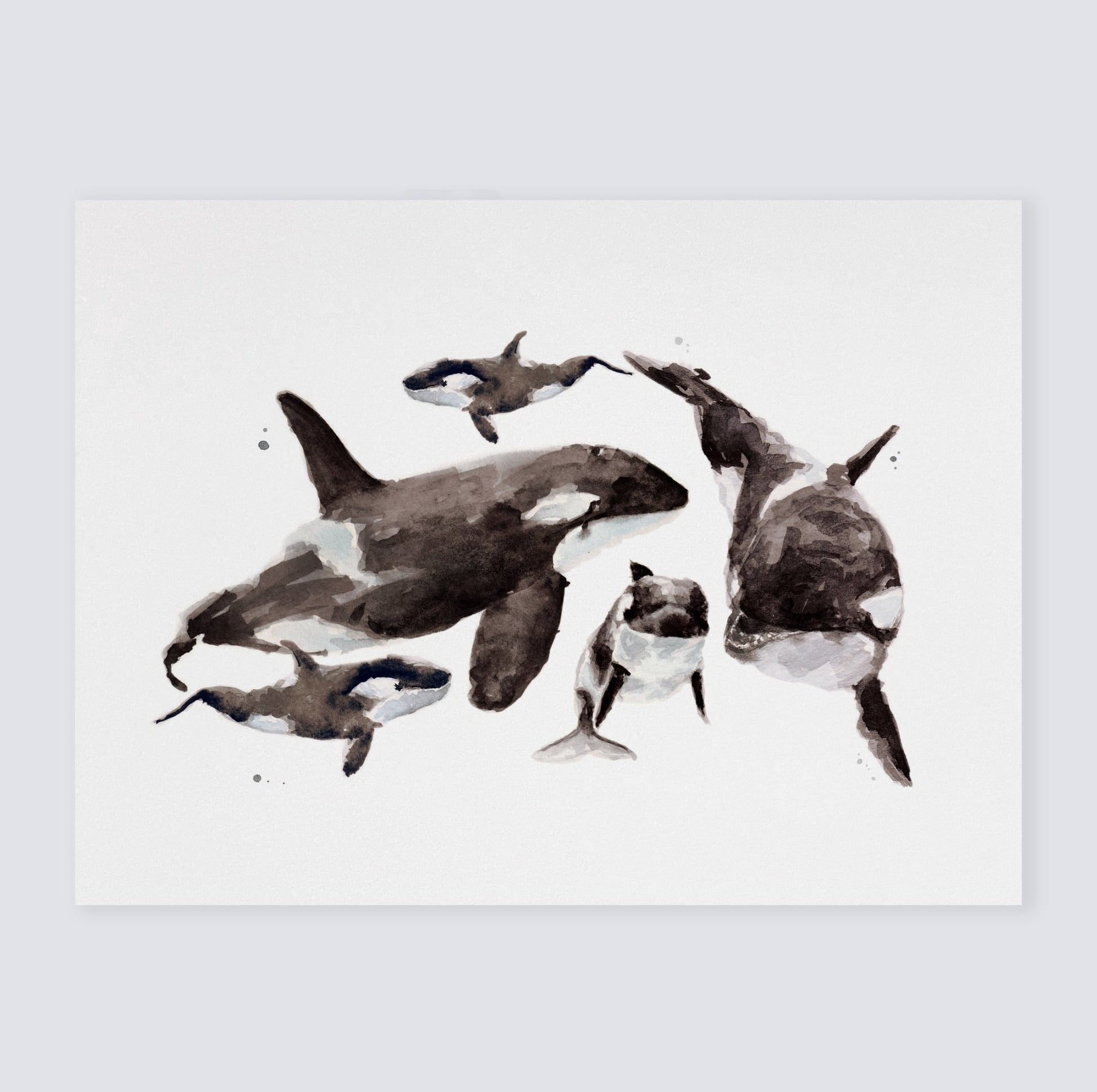In this detailed watercolor painting, we see a lively family of five killer whales, gracefully positioned against a light gray square background. The artwork is horizontally oriented, with the colors primarily consisting of blotchy blacks, whites, and various shades of gray, skillfully blending to create a realistic yet artistic depiction of the orcas. The largest killer whale, positioned on the right, faces forward with its tail visible curving behind it. To its left, another adult orca faces towards the largest whale, its nose pointed rightward. Above this second whale, a baby killer whale is oriented leftward, adding a playful touch to the composition. Beneath the head of the leftward-facing adult, another small orca swims towards the viewer, enhancing the dynamic interplay of directions. Finally, near the tail of the left-facing adult, a third baby orca completes the family group. Interspersed around the whales are small, round gray bubbles, adding to the depth and lively nature of the scene. The professional craftsmanship of varying brushstrokes and shades brings this serene portrayal of killer whales to life, suggesting a harmonious underwater dance.